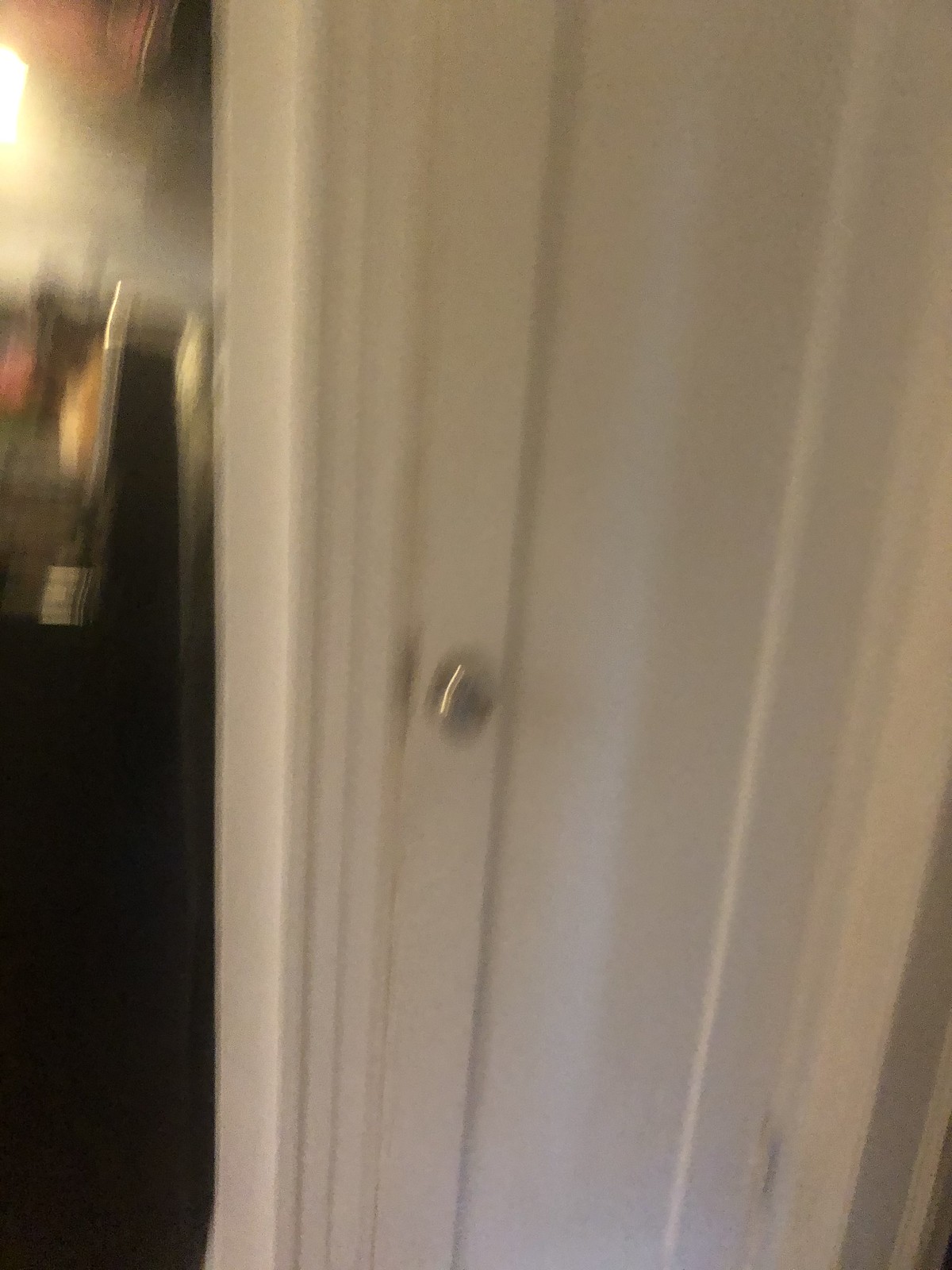The image, though blurry, depicts a tall white door with a silver handle, slightly ajar. To the left of the door, partially visible, is a piece of furniture placed against a white wall. A clothing item, appearing to be brownish-pink in color, hangs nearby. Adjacent to the door is a dark wooden stand adorned with indistinguishable items. The white door seems to lead to another room in the house or area.